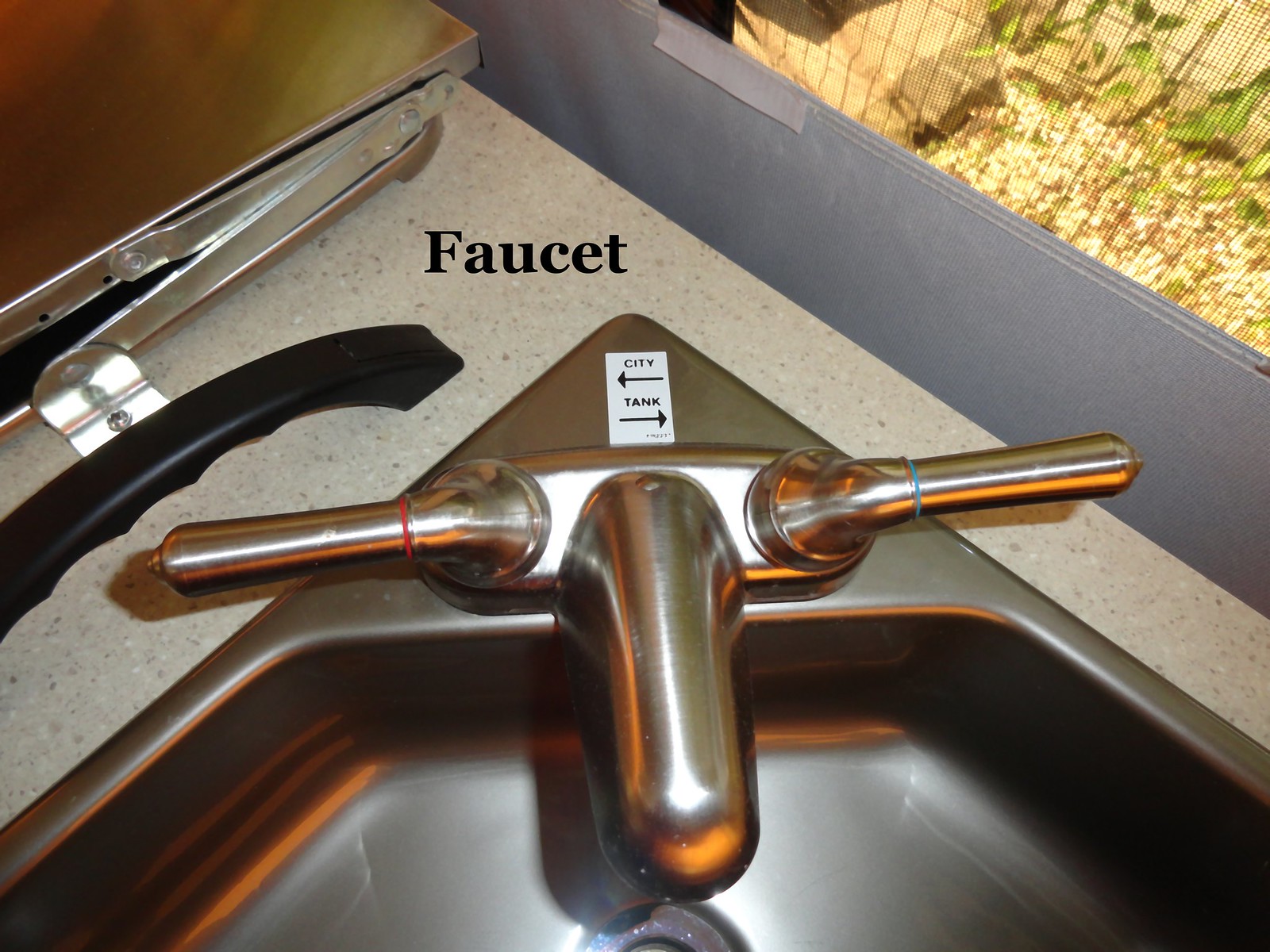This image depicts a kitchen sink set into a laminate countertop that has a pinkish-gray base with white and gray flecks. The sink itself is shallow and appears to be made of metal with a bronze or copper color reflection. The faucet is plasticky silver with two cylindrical handles: the left handle has a red band indicating hot water, while the right handle has a blue band for cold water. At the base of the faucet, there is a white sticker with black letters that says "city" with an arrow pointing to the left, and "tank" with an arrow pointing to the right. The counter also features some indistinct shiny chrome objects and a black plastic item. Situated behind the sink, on the right wall, there's a mysterious structure that looks like a cage containing vegetation and brown dirt. This setup appears to be inside a structure, possibly resembling the interior of a tent, and overall it looks new and unused.